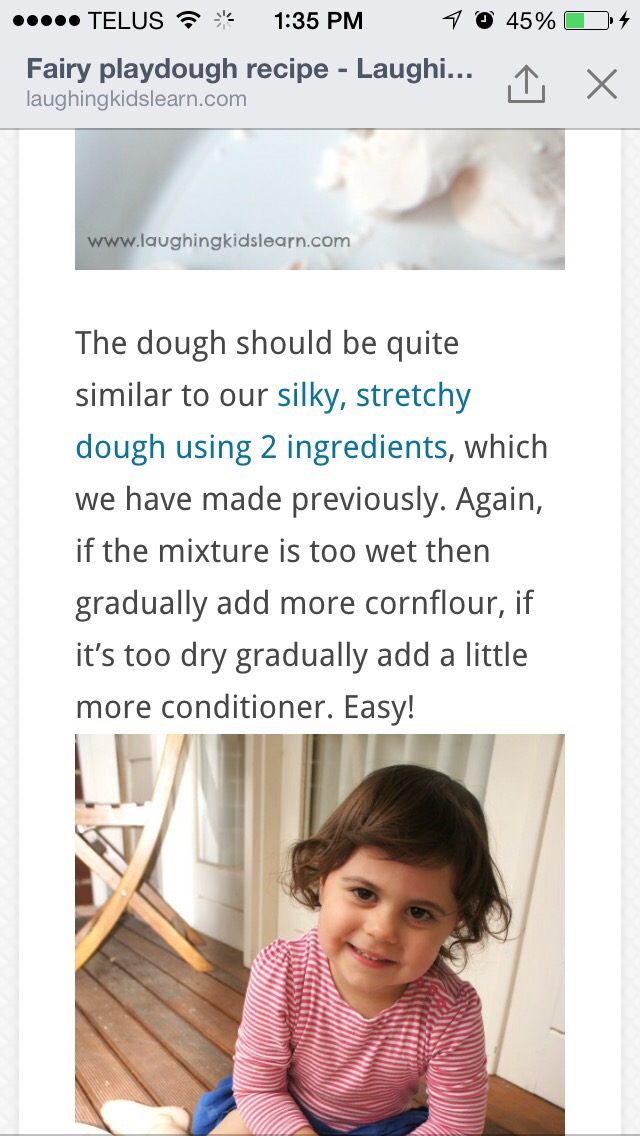The image is a screenshot taken from an iPhone at 1:35 PM, with the battery at 45% and full signal bars. The title of the article displayed is "Fairy Play-Doh Recipe," sourced from the website laughingkidslearn.com. The website has a white background and the text reads: "The dough should be quite similar to our silky, stretchy dough using two ingredients, which we have made previously. Again, if the mixture is too wet then gradually add more cornflour. If it's too dry, gradually add a little more conditioner. Easy!" Below this text, there is a photo of a young girl, approximately two years old, with short brown hair. She is wearing a long-sleeved, red and white horizontally striped shirt and blue bottoms, sitting on a wooden deck or patio. The overall presentation of the image focuses on the Play-Doh recipe and instructions, accompanied by the picture of the smiling child.